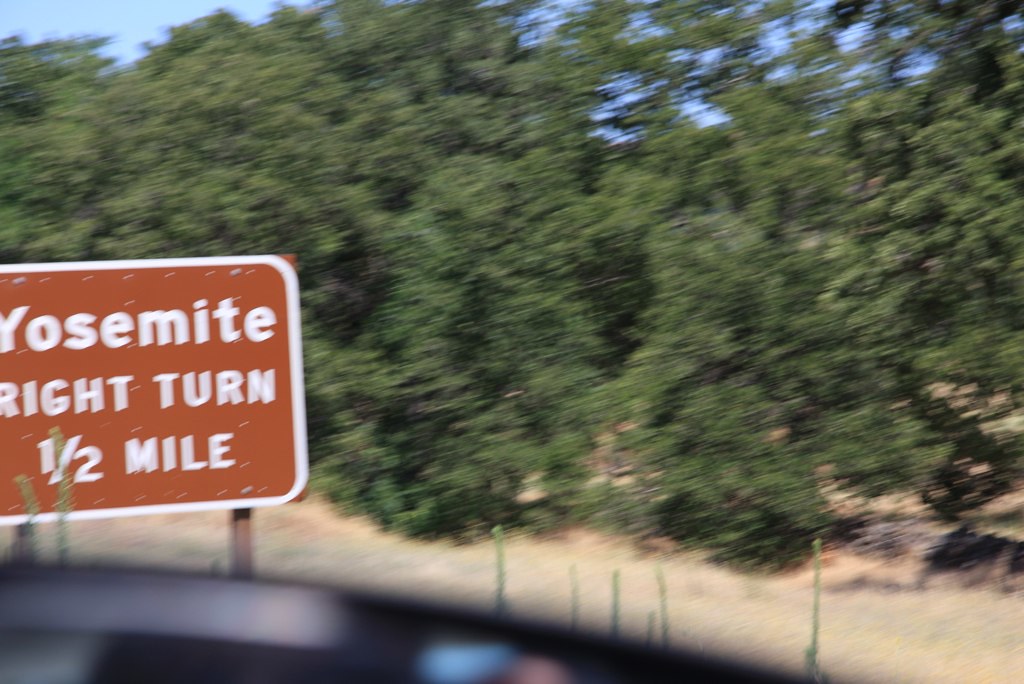This somewhat blurry photograph appears to have been taken from inside a moving car, revealing a partial view of the dashboard in the bottom left corner. The image captures a scene alongside a highway, dominated by lush, green trees that stretch across the background beneath a clear blue sky. Positioned on the left side of the photo, a prominent road sign indicates a right turn for Yosemite in half a mile. This brown sign with white text is supported by two wooden poles. The roadside scenery includes a glimpse of either a fence or additional greenery. The blur suggests the photograph was taken hastily, focusing primarily on capturing the directional sign amidst the natural setting.